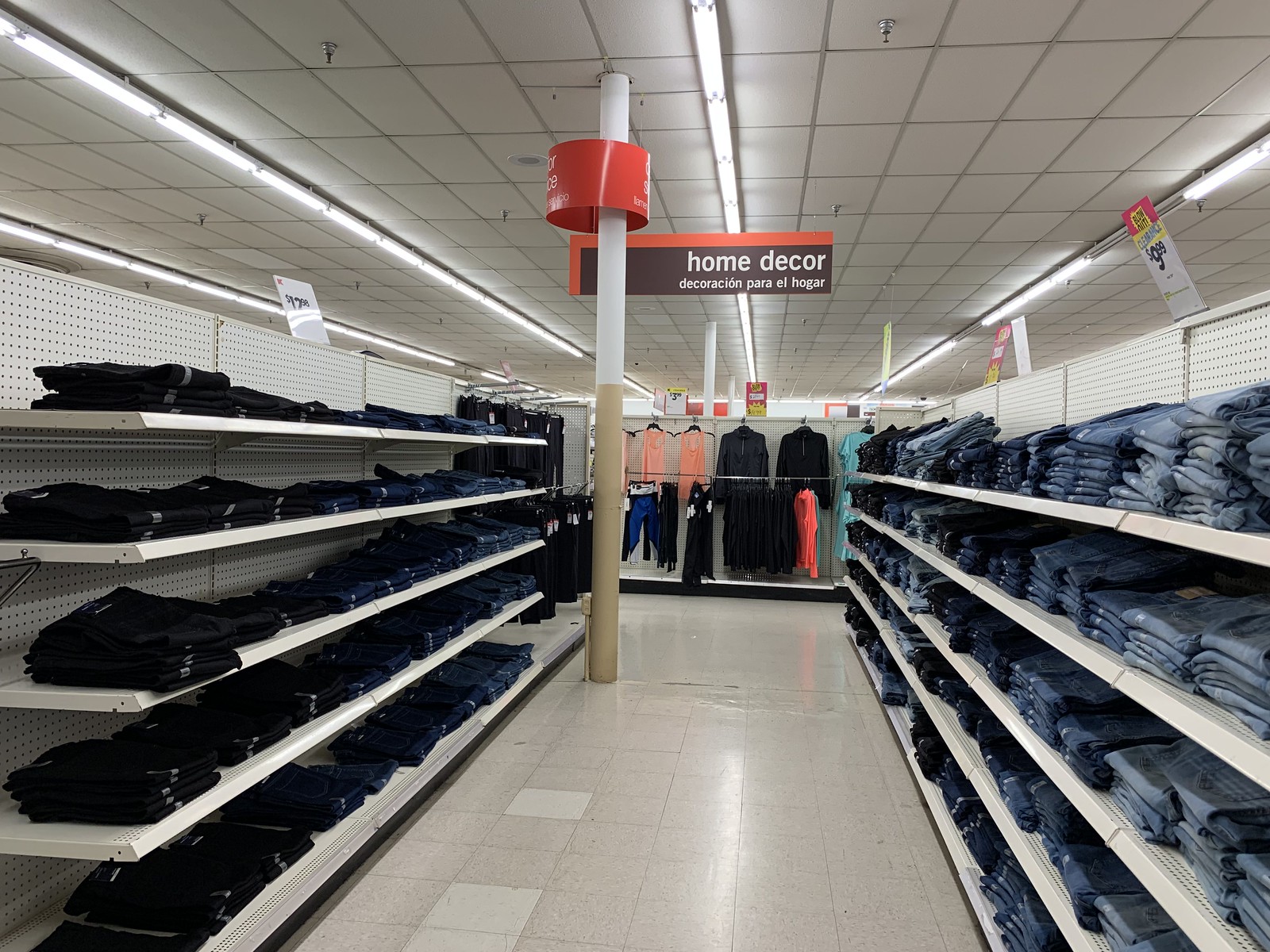This image captures the interior of a large department store from a first-person viewpoint, emphasizing an aisle surrounded by display shelves filled with neatly folded jeans. The aisle is flanked by white display shelves, with the left side holding black and denim jeans, while the right side features a fuller stock of lighter denim jeans. Above the aisle, fluorescent tube lighting is installed across a ceiling grid. A prominent white and brown pole extends from the floor to the ceiling, supporting a red and brown sign that reads "Home Decor" and beneath it, the text "Decoración para el hogar" in Spanish. Tiled floors with a mix of whiter and darker polished tiles stretch ahead. The pole also features price signs attached to the top shelf. Near the ceiling, a cylindrical sign is partially visible, suggesting additional information not entirely readable from the captured angle.